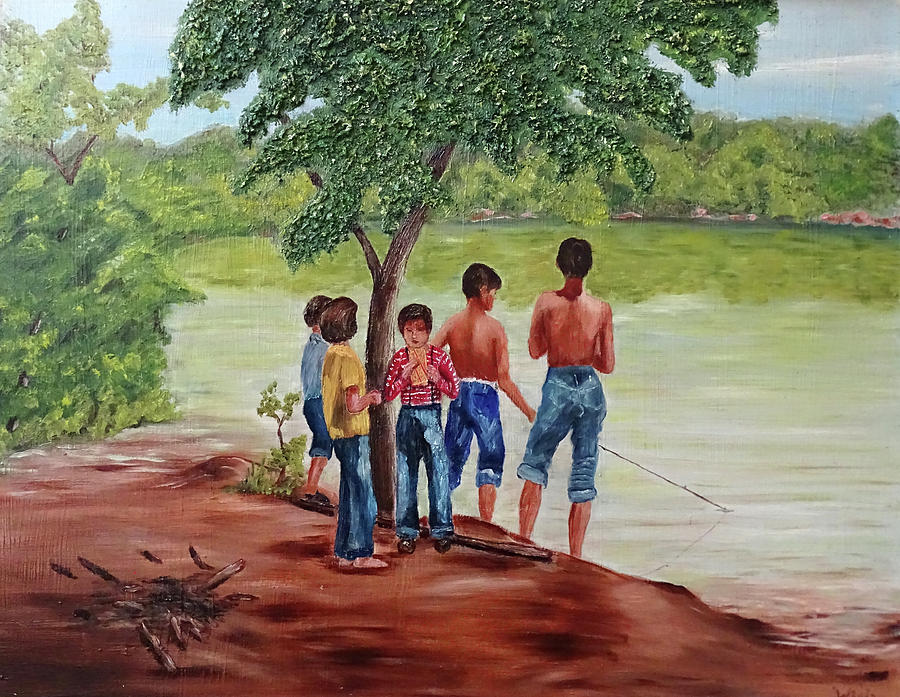This watercolor painting captures a serene summertime adventure featuring five young boys standing on the edge of a small lake or river, beneath the shade of a vibrant, green tree. The group is depicted on a brown and muddy shoreline, where remnants of a burnt campfire and scattered wood are visible. Two of the shirtless boys, wearing rolled-up blue jeans, are engaged in fishing, with one holding a fishing pole over the water. The other three boys stand nearby, each wearing blue jeans and colorful shirts: one in a red and white striped shirt with suspenders, another in a yellow shirt, and the last in a light blue shirt. The reflective water mirrors the surrounding lush greenery and the partly cloudy sky, enhancing the painting's natural, tranquil atmosphere. The scene, reminiscent of a carefree day from the 1980s, is characterized by its green and brown color palette, emphasizing the vibrant and earthy tones of the setting.